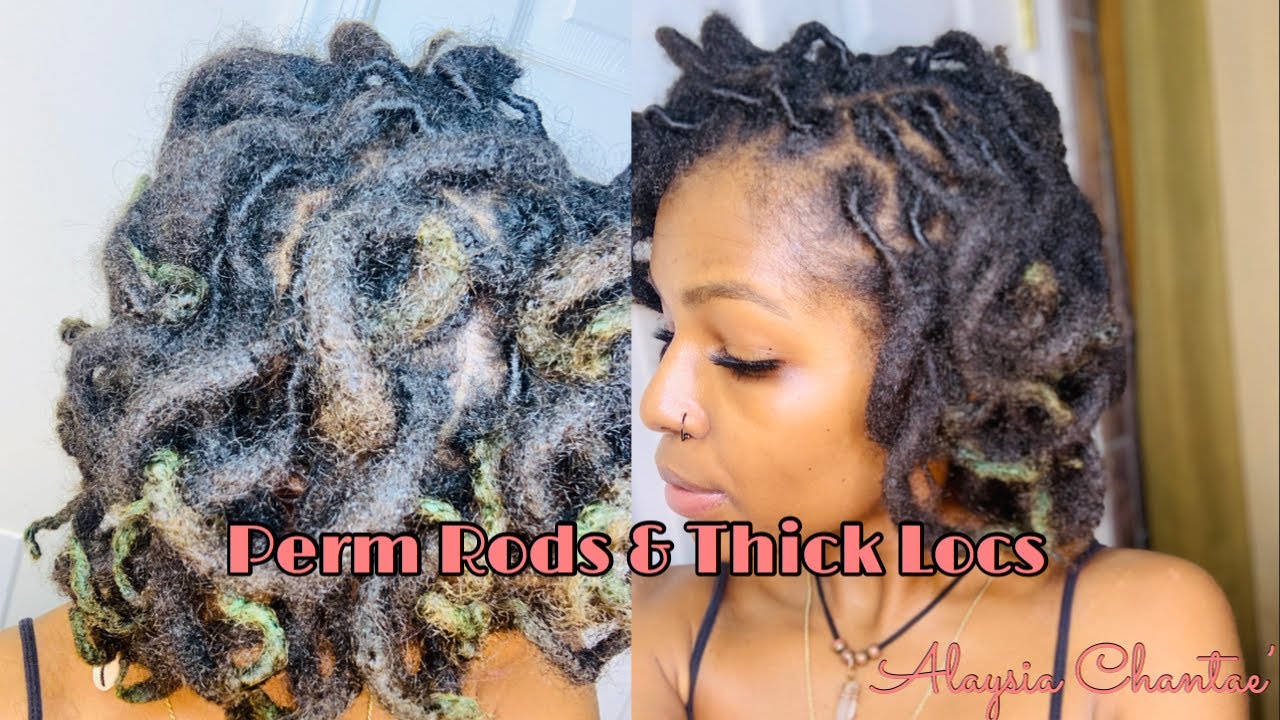The image is an advertisement for a hairstyling service called "Perm Rods and Thick Locks," featuring before-and-after photos of a woman with thick dreadlocks, which have a slightly green color hint, possibly due to permanent coloring. The text at the bottom confirms this service and the artist's name, Alessia Shante. The woman depicted is adorned with two necklaces and a nose ring, and her thick eyelashes enhance her natural beauty. The right side of the image subtly shows a door in the background, adding a naturalistic, unprofessional feel to the photographs, as if they were candid shots taken with a regular camera.